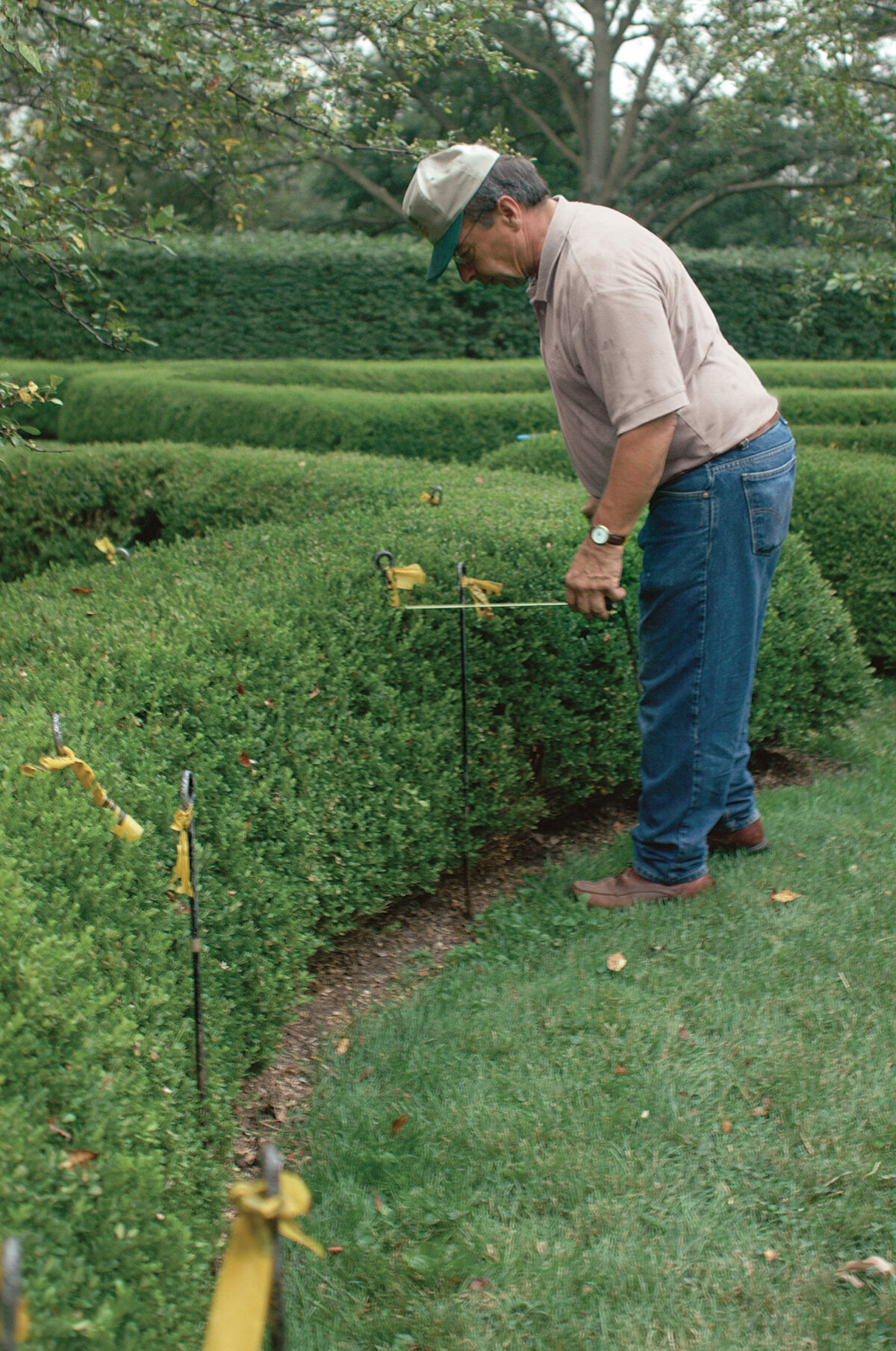This color photograph captures a man meticulously working in an ornate garden with lush, manicured greenery all around. Positioned to the right, the man is dressed in a short-sleeved gray tennis shirt paired with blue jeans, a brown belt, brown shoes, and a brown watch. He sports a gray hat with a green brim and glasses. He is leaning over towards a neatly trimmed boxwood hedge, holding a light-colored tape measure or similar stick-like device, seemingly measuring the distance from the front of the hedge to a farther point.

The garden itself is a display of horticultural excellence with vibrant green grass beneath the man's feet, and well-maintained shrubs and hedges forming various shapes and sizes. The hedges extend from the lower left, curve behind the man, and create an ornamental landscape, including some waist-high round hedges and a taller hedge resembling a verdant wall. Little poles with yellow ribbons are set in front of the hedges.

In the background, there are more hedges, lush foliage, and a tall tree with slender branches and small green leaves, contributing to the tranquil and meticulously cared-for atmosphere of the garden. This serene, green haven is further accented by scattered yellow leaves and various types of shrubbery, adding layers of natural beauty to the scene.